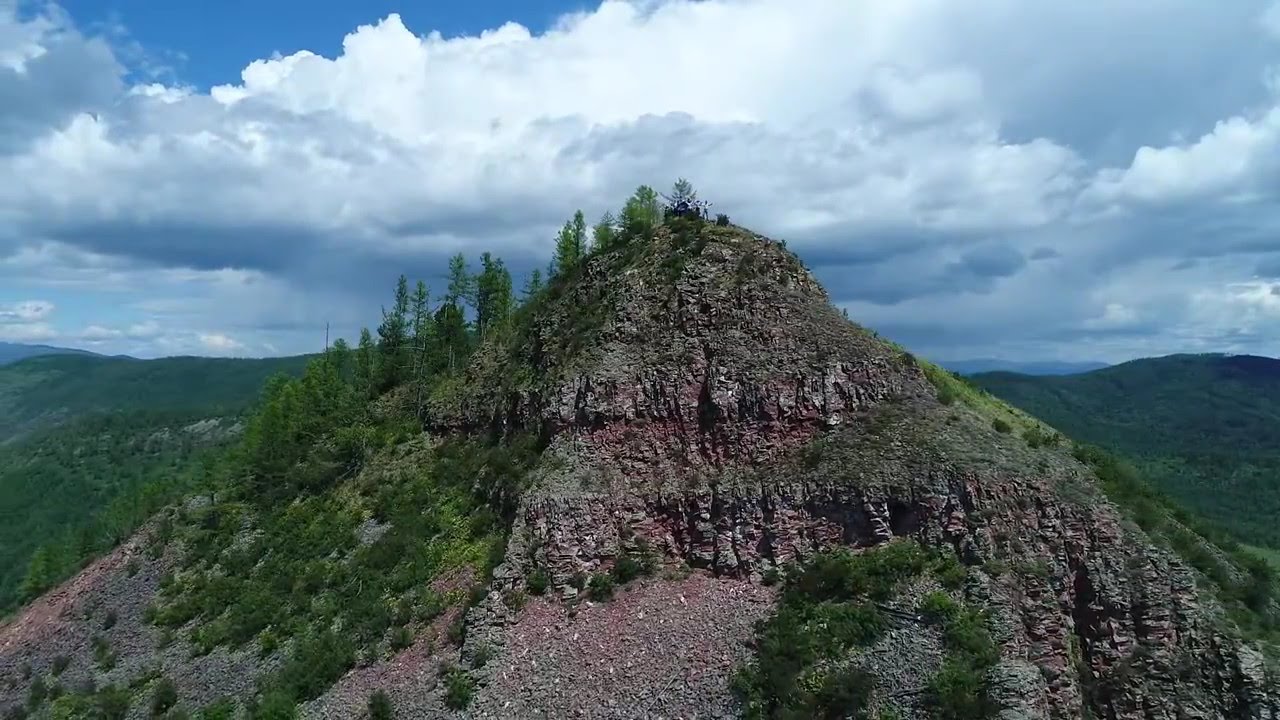The photograph captures an outdoor nature scene on an overcast day with a sliver of blue sky visible amidst thick, heavy white clouds. The upper half of the image is dominated by a sky full of large, fluffy white clouds, with their undersides tinged a deep blue-gray. Central to the composition is a modest mountain or large hill, predominantly composed of bare, rocky surfaces in shades of brown and gray. The lower section of the mountain features dull, reddish-brown dirt with scattered stones and minimal vegetation. However, the upper sections are adorned with green pine trees, grass, and scrub brush. The sheer cliffs of the mountain exhibit deep indentations, showcasing fallen stones. Flanking this central peak are rolling, tree-covered hills that stretch towards the horizon. The overall atmosphere is that of a serene and rugged landscape, framed by the contrasting colors of the earth and sky.